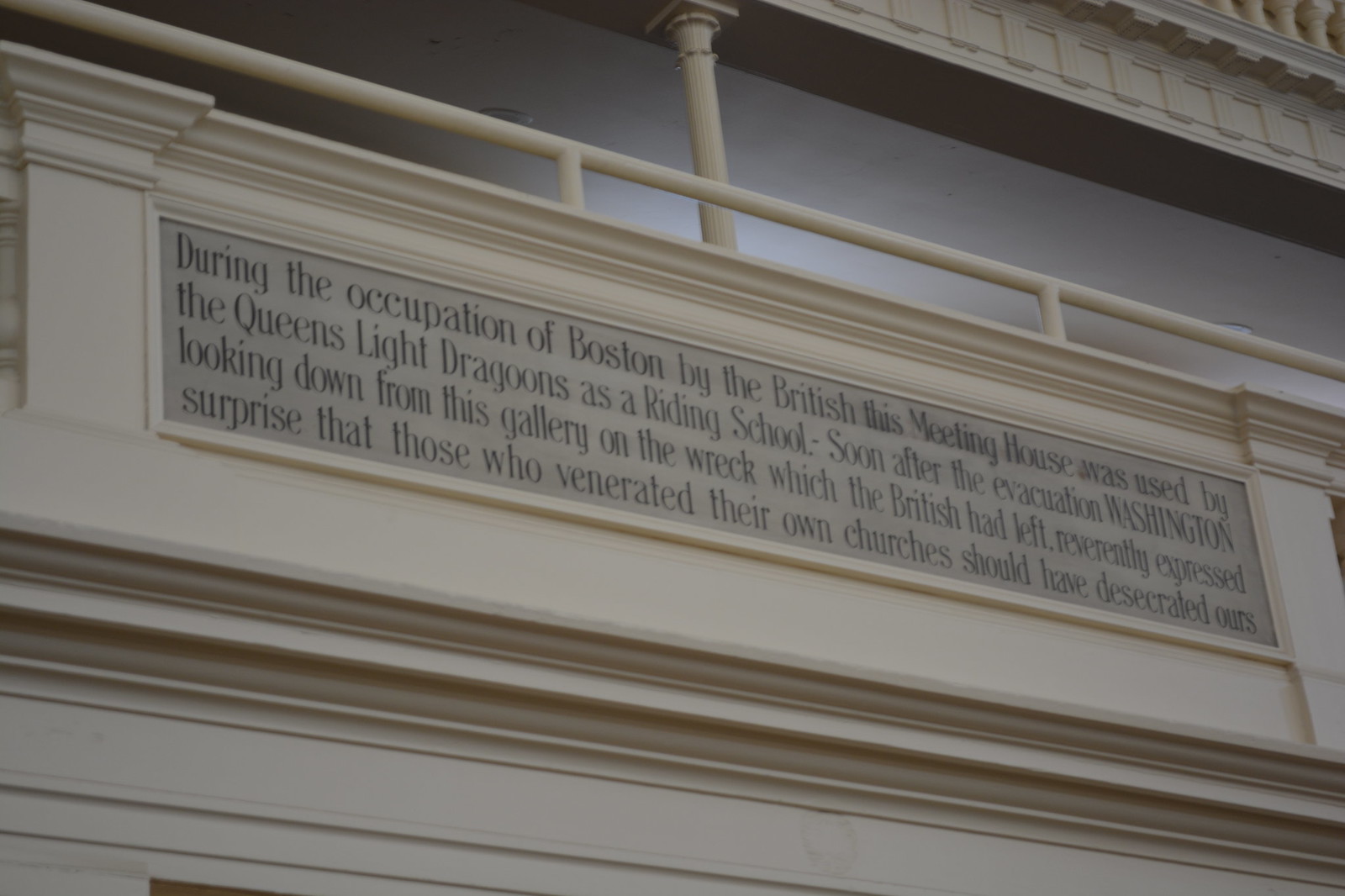The image depicts a section of a multi-story white building, focusing on an interior plaque mounted on a silver background with black lettering. The plaque, located on what appears to be the first or second floor, is an important historical marker. It states: "During the occupation of Boston by the British, this meeting house was used by the Queen's Light Dragoons as a writing school. Soon after the evacuation, Washington, looking down from this gallery on the wreck which the British had left, reverently expressed surprise that those who venerated their own churches should have desecrated ours."

The setting includes architectural details like a railing across the top of a wall and a decorative pillar supporting the ceiling from the upper floor, suggesting a sophisticated interior. The text on the plaque is made to look handwritten but is clearly painted or printed, adding to the historical ambiance of the setting. The predominant color in the rest of the image is white, further highlighting the significance of the plaque.